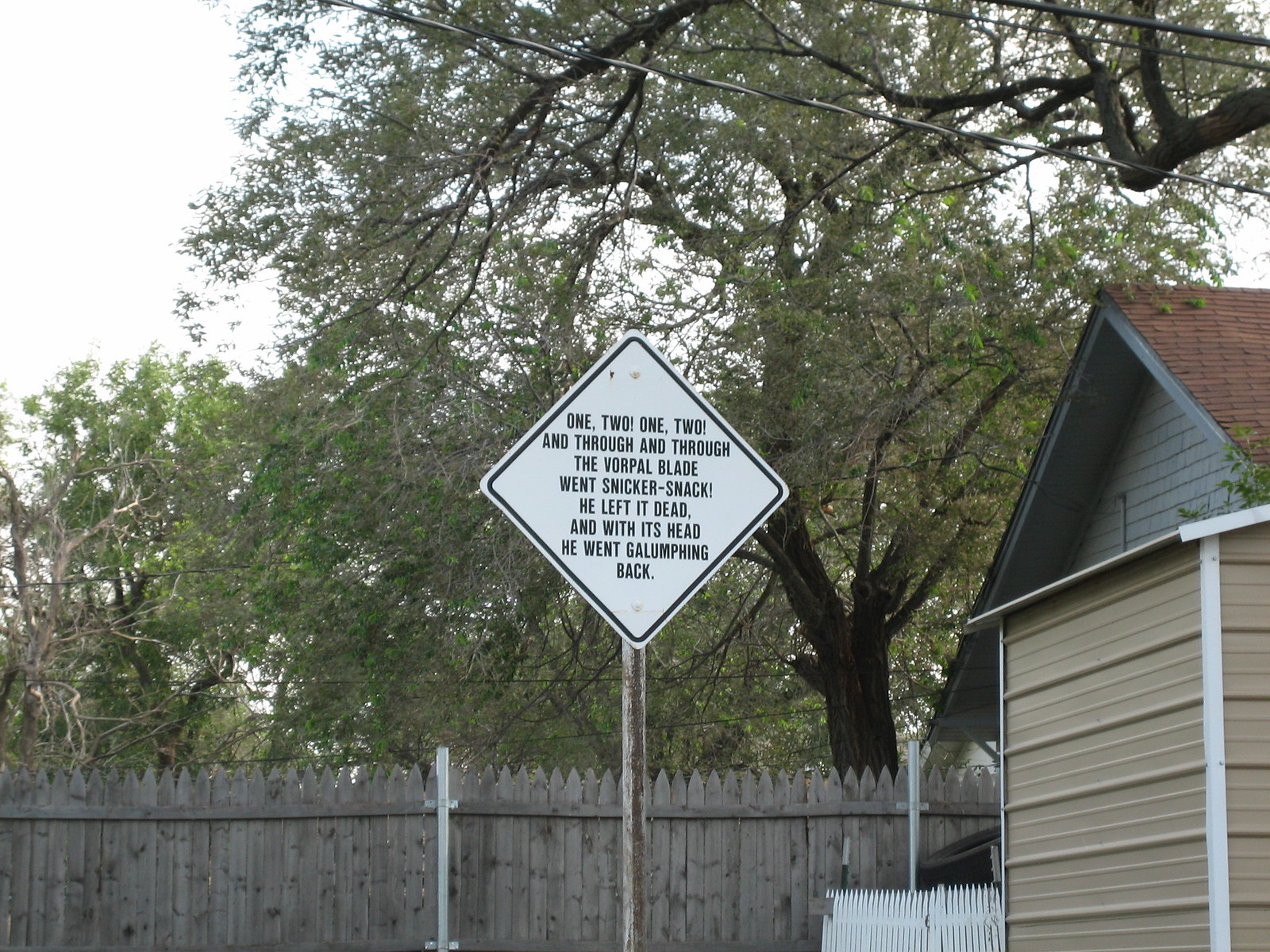The image depicts an outdoor scene in a backyard on an overcast day. At the center, there is a weathered triangular road sign mounted on a faded wooden pole. The off-white sign, bordered in black, features a whimsical poem in black text: "One, two! One, two! And through and through, The vorpal blade went snicker-snack! He left it dead, and with its head He went galumphing back." The sign, despite its peculiar content, resembles a typical road sign but conveys a passage from Lewis Carroll's "Jabberwocky."

In the background, slightly to the right, stands a tan-colored metal shed with white corners and a white roof. Adjacent to the shed is a small white wooden picket fence. To the far right, part of the roof of a gray house with red shingles is visible. Stretching across the image is a power line running diagonally from the center to the top-right corner. Additionally, there is a weathered wooden picket fence with a spiky top section on the left side, extending into the background where large, tall trees are prominent.